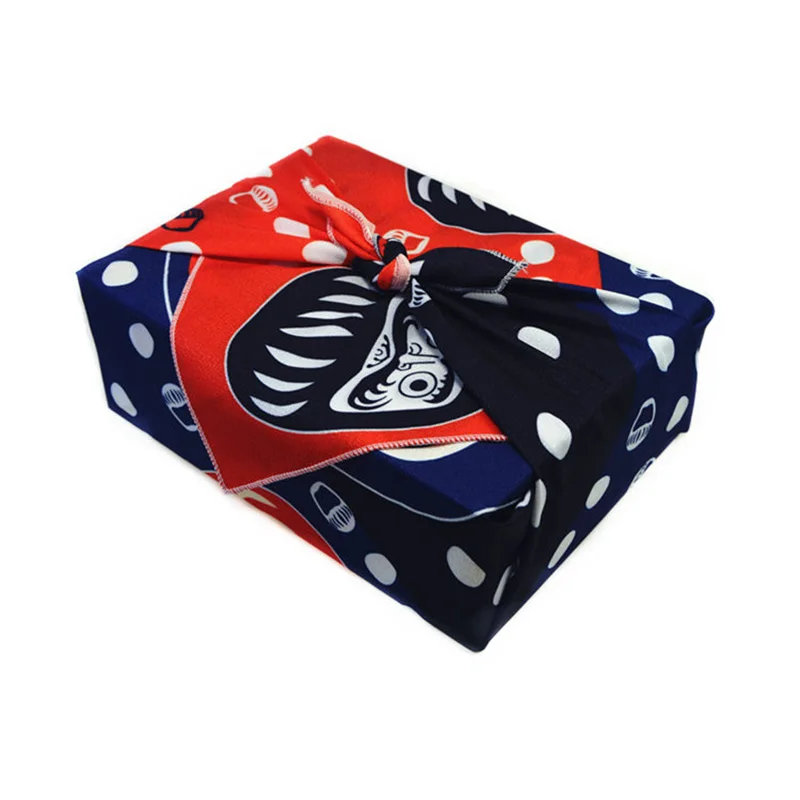The image depicts a rectangular box, resembling a shoebox, entirely wrapped in a colorful fabric. The fabric is a patchwork of navy blue, black, white, and red sections. The navy blue and black portions are decorated with white polka dots, while the striking red section features a repeated white demon-like face motif, each missing eyes. The fabric is carefully tied into a knot at the top of the box, with some edges of the red fabric sewn around the perimeter, giving it a finished look. There is a prominent black symbol enclosed in a red border at the top center of the box, adding a unique touch to the overall wrapping. The image is set against a stark white background, which emphasizes the vibrant colors and intricate patterns of the wrapped box.